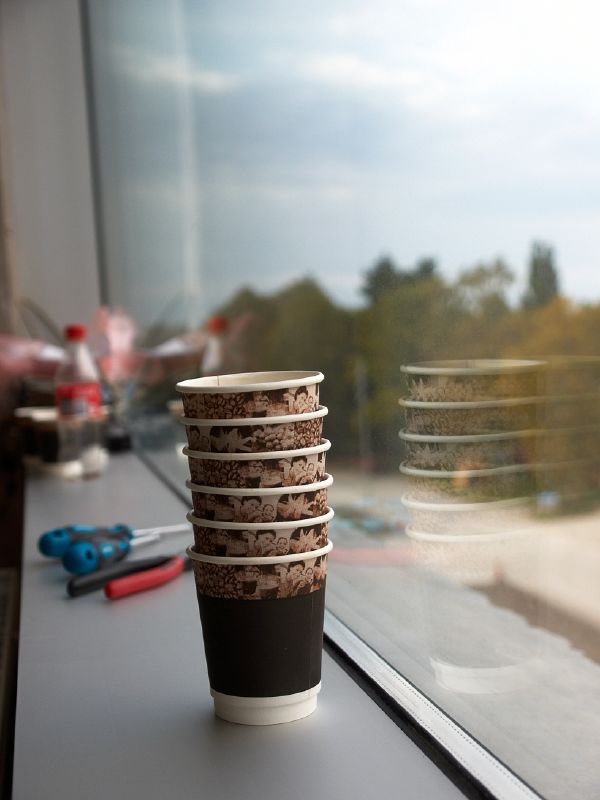In this portrait-style photograph, six one-time-use brown coffee cups, resembling those found at hotels or coffee shops like Starbucks or Tim Hortons, are stacked neatly inside one another on a windowsill. The bottom cup features a black hot sleeve for insulation, and each cup is adorned with old-style, blurry face designs around the rim. Situated to the right of the photo, the windowsill overlooks a serene, blurry forest blending shades of green and orange. The sky above the forest is a vivid blue with scattered clouds, through which the sunlight peeks, illuminating parts of the scene. Reflected in the windowpane are the cups themselves, and the shelf they rest on. Also visible are tools, including two blue and black-handled steel screwdrivers and a pair of orange and black pliers—possibly a wire cutter—blurred in the background. An empty red plastic Coca-Cola bottle also sits farther back on the shelf, contributing to the photo’s layered composition.